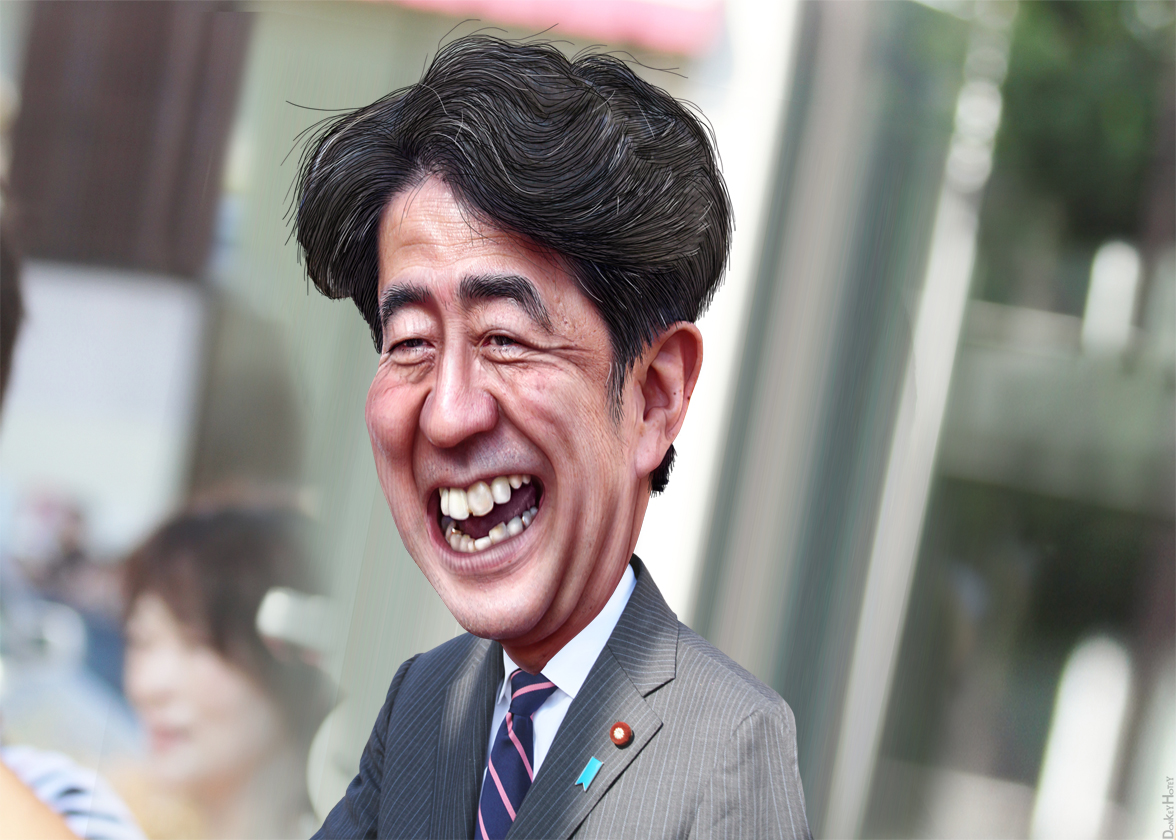This highly detailed caricature photograph showcases a middle-aged Asian man with an exaggerated, oversized head rendered in cartoonish style. His thick, dark black hair, with hints of gray, is parted slightly on the right. He exudes a jovial energy, with crinkled eyes and an open-mouthed laugh that reveals imperfect teeth. His exaggerated facial features, particularly the smile and eyes, are cartoon-like with distinct coloring and outlining.

He wears a light gray suit jacket accented with thin pinstripes, a crisp white button-down shirt, and a navy or purple tie featuring gold or thin pink stripes. On his left lapel, he has a prominent red round button and a light blue ribbon-style pin. The man is photographed at a three-quarter angle facing left. The background, though blurred, suggests an outdoor setting near a building with additional blurred figures, including an indistinct Asian woman with medium-length hair on the lower left. The entire image is heavily filtered to enhance the caricature effect, giving it a bobble-head appearance.